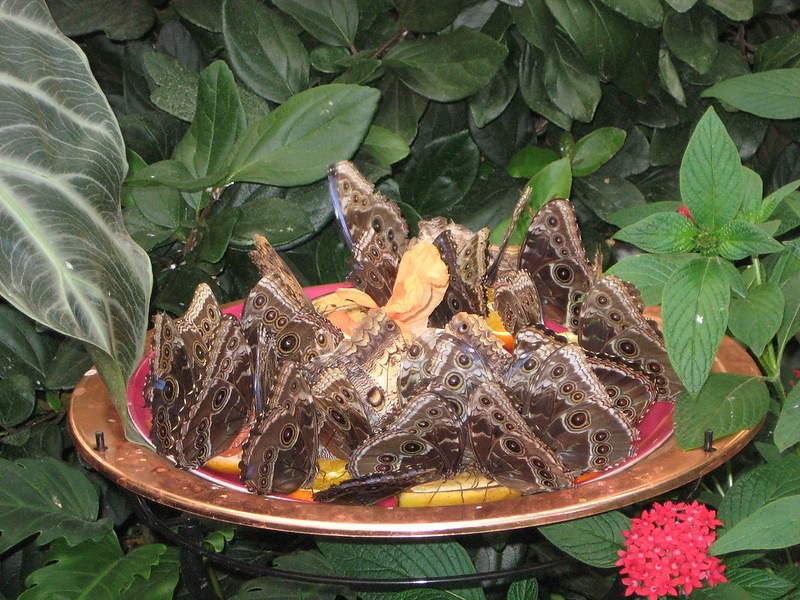In this detailed photograph, we see a captivating scene set against a lush backdrop of various green leaves, ranging from dark to light shades, typical of a diverse array of plants and bushes. The composition is horizontally framed, with a striking large green leaf in the top left corner and vibrant red blossoms in the bottom right adding pops of color. Central to the image, nestled among the foliage, is a brass dish or bowl held up by a black metal stand. This dish is the focal point, attracting around 20 butterflies distinguished by their dark brown wings adorned with black, brown, and white circle patterns. A unique butterfly with slightly different markings can be seen in the center. The butterflies all appear to be flocking to the dish, which contains a mix of yellow and red items—possibly flowers or food—adding to the allure of the scene. Their wings are predominantly upright, showcasing intricate patterns, with the occasional glimpse of delicate legs. This captivating moment captures the fluttering congregation in mid-landing around the enticing center of attraction within the verdant setting.